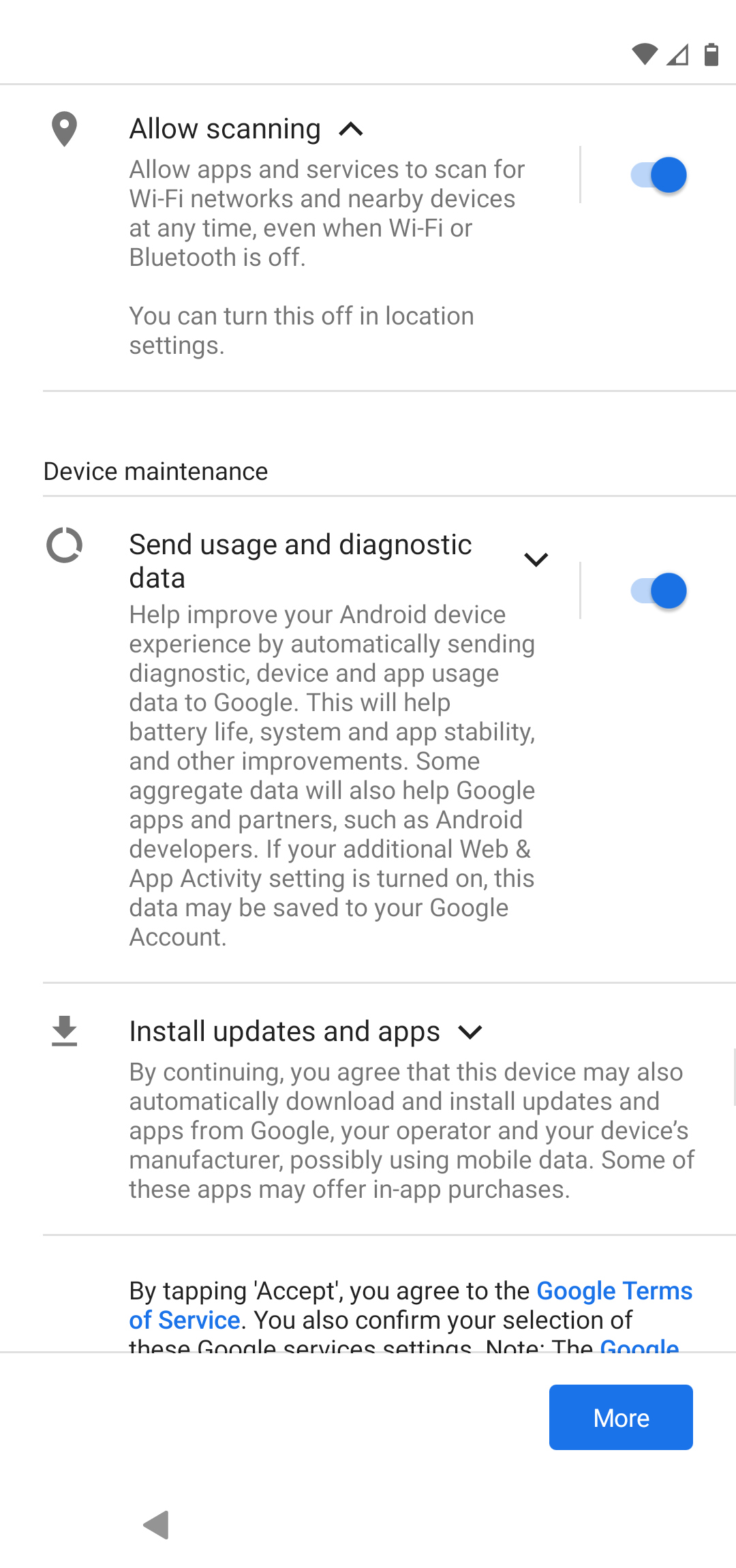This photograph captures a smartphone's settings page with several toggles and informational prompts. The top of the screen includes standard status indicators such as a Wi-Fi icon, a triangular cellular signal icon with a partially filled section, and a battery icon that is approximately three-fourths full, confirming the device is indeed a phone.

The first setting displayed is about location services, illustrated by a map pin icon. It reads "Allow scanning," with a description stating: "Allow apps and services to scan for Wi-Fi networks and nearby devices at any time, even when Wi-Fi or Bluetooth is off. You can turn this off in location settings." This option is activated, as indicated by the blue toggle switch.

Following this is the "Device maintenance" section, marked with a circular icon. It states, "Send usage and diagnostic data," with further details: "Help improve your Android device experience by automatically sending diagnostic device and app usage data to Google. This will help battery life, system, and app stability, and other improvements. Some aggregate data will also help Google apps and partners, such as Android developers. If your additional web and app activity setting is turned on, this data may be saved to your Google account." This feature is also enabled, as shown by the blue toggle.

The final setting relates to updates and downloads, symbolized by a download icon. It reads "Install updates and apps" with the explanation: "By continuing, you agree that this device may also automatically download and install updates and apps from Google, your device’s manufacturer, possibly using mobile data. Some of these apps may offer in-app purchases." This section does not feature a toggle option and remains unticked.

At the bottom of the screen, there's a message: "By tapping accept, you agree to the Google Terms of Service. You also confirm your selection of these Google services settings. Note the Google…" with the text truncating, followed by a blue button labeled "more" suggesting additional information or options can be accessed.